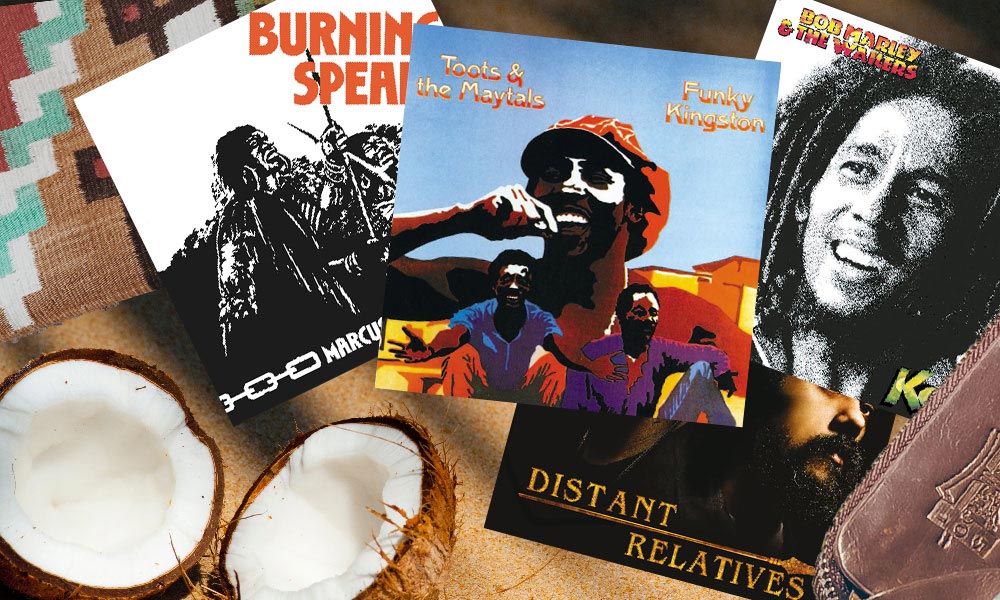This overhead photograph reveals a striking display of vinyl record covers set against a sandy backdrop. In the upper left corner lies a vibrant woven tapestry featuring shades of white, mint green, red, light brown, and dark brown. Anchoring the bottom left is a halved coconut, its brown, fibrous shell contrasting with the smooth white meat inside. The focal point consists of four prominent album covers. On the left is "Burning Spear," partially obscured, showcasing a Native American chief illustration and the text in orange on a white background, with hints of silhouetted human figures and additional concealed text. The central album, "Funky Kingston" by Toots and the Maytals, bursts with color, depicting three African American men against a vivid palette of black, white, purple, blue, red, orange, yellow, and brown. To the right, a black and white album cover portrays the iconic Bob Marley, with his name and "The Wailers" inscribed at the top. Partially visible beneath it is another album, "Distant Relatives," featuring a black man with black facial hair and the title in gold lettering. The composition of the scene beautifully melds musical nostalgia with tropical and earthy elements.